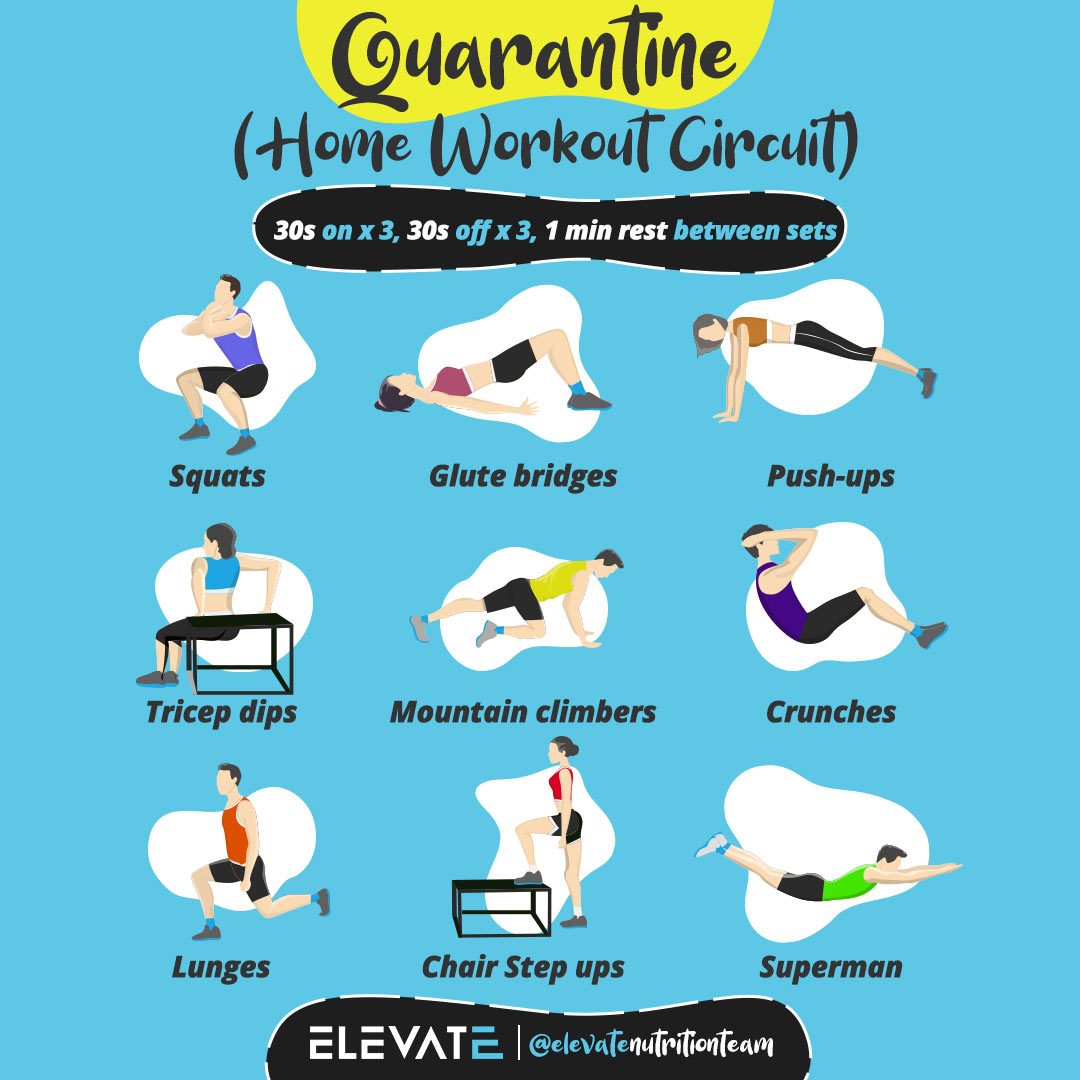The image depicts a brightly colored workout routine poster set against a blue background. At the top, against a mustard yellow bubble, the word "quarantine" is written in a stylish, feminine font, followed by "home workout circuit" in parentheses. Below, in a black bubble with white and blue text, instructions detail: "30 seconds on x3, 30 seconds off x3, 1 minute rest between sets."

The poster showcases three rows of cartoon-like illustrations representing different exercises. Each row features three individual exercises:

1. **Top Row:** 
    - A man in a purple tank top and black shorts performing squats.
    - A woman in a maroon tank top and black shorts doing glute bridges.
    - A person in a brown tank top and black capri pants executing push-ups.
2. **Second Row:**
    - An individual in a blue top and black pants performing tricep dips on a table.
    - A person in a green tank top and black pants doing mountain climbers.
    - An individual in a purple tank top and black pants doing crunches.
3. **Bottom Row:**
    - Someone in an orange tank top and black pants engaged in lunges.
    - An individual in a red tank top and black shorts doing chair step-ups.
    - A person in a green tank top and black shorts doing the Superman exercise.

Each exercise is labeled underneath its corresponding illustration. At the bottom of the poster, in a black bubble with white and blue lettering, it reads: "elevate @elevatenutrition.com."